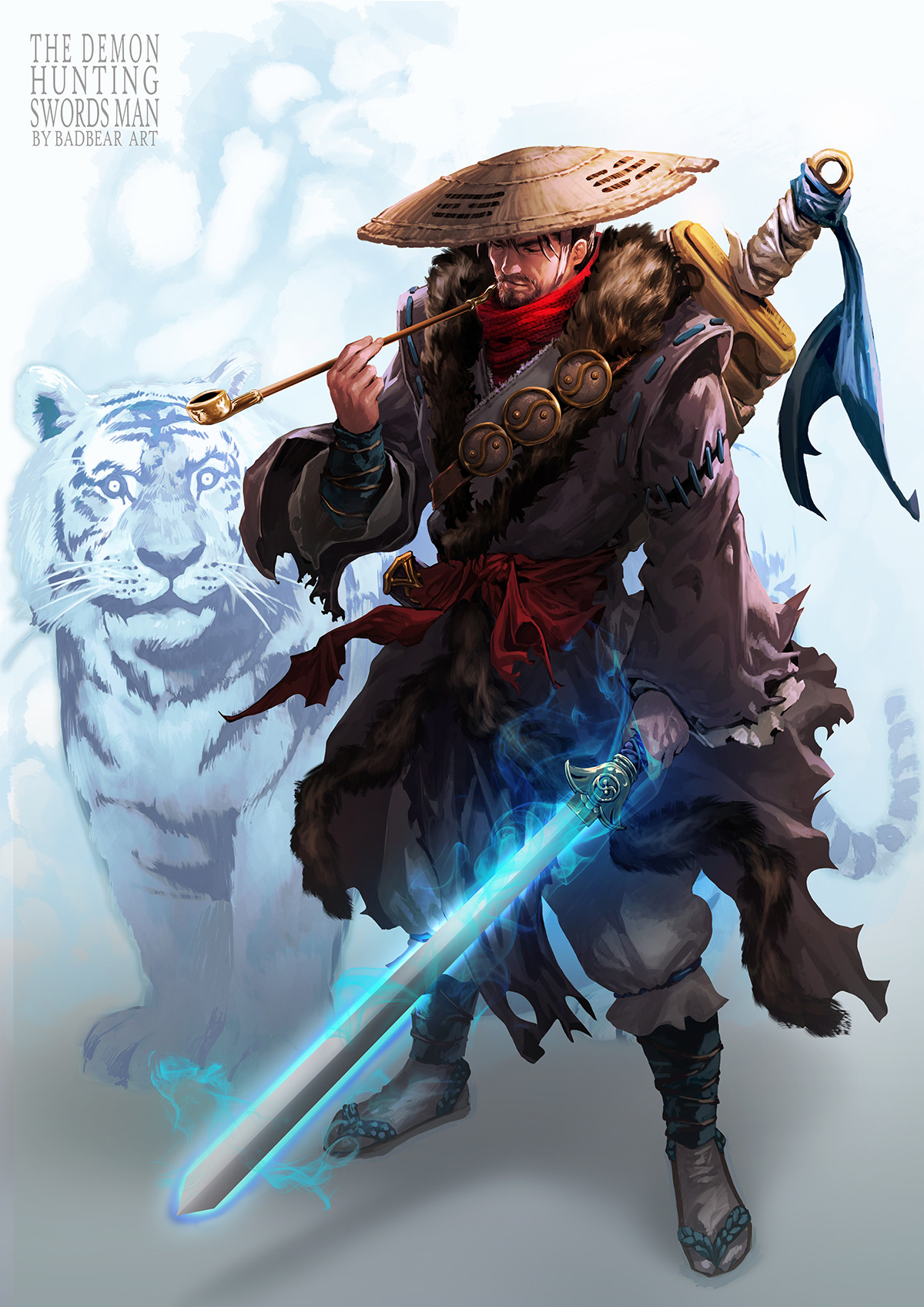This digital artwork, possibly inspired by video game aesthetics, portrays an enigmatic character known as the "Demon-Hunting Swordsman" by Bad Bear Art. The scene features an Oriental warrior clad in cold-weather attire, including a distinctive flat hat resembling those worn in Japan or Southeast Asia, and gray boots tinged with greenish-blue hues. The warrior wields an ethereal, blue-glowing broadsword in his left hand, while a second, intricately detailed saber with a gold and white handle and a small blue flag is sheathed across his back. Additional fighting implements are strapped across his chest in a leather scabbard adorned with round brass plates. The lone warrior is also depicted smoking a long, brass opium pipe, adding to his mysterious persona.

In the background looms the shadowy silhouette of a tiger, almost spectral in its presence, featuring white fur with distinctive black markings. This ghostly companion appears vigilant, peeking around a corner and standing by the warrior's side. The artwork's upper left corner bears the title "The Demon-Hunting Swordsman" along with the artist's signature, Bad Bear Art.